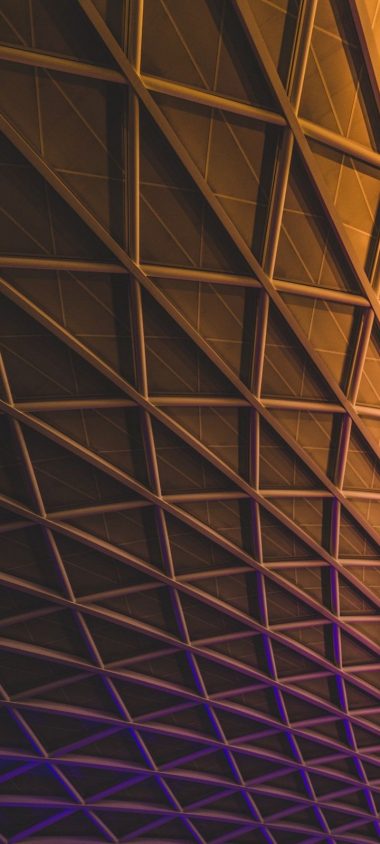The image features a close-up view of an architectural structure, likely a ceiling or the side of a building, characterized by an intricate steel latticework. The composition showcases a grid with cross beams extending diagonally from the upper left to the lower right corner, creating a series of triangular patterns reminiscent of Sierpinski's triangle. This pattern appears larger at the top and diminishes in size towards the bottom, with a subtle curvature that adds to its complexity. Light plays a significant role in altering the appearance of the structure: the lower portion of the image is bathed in a rich purple hue, transitioning to a warm amber tone at the top with a gradient effect. The texture of the surface also reveals squares formed by intersecting vertical and horizontal lines, each bisected by diagonal bars, contributing to a detailed and dynamic visual composition that evokes the geometric intricacies of the Epcot Center ball.